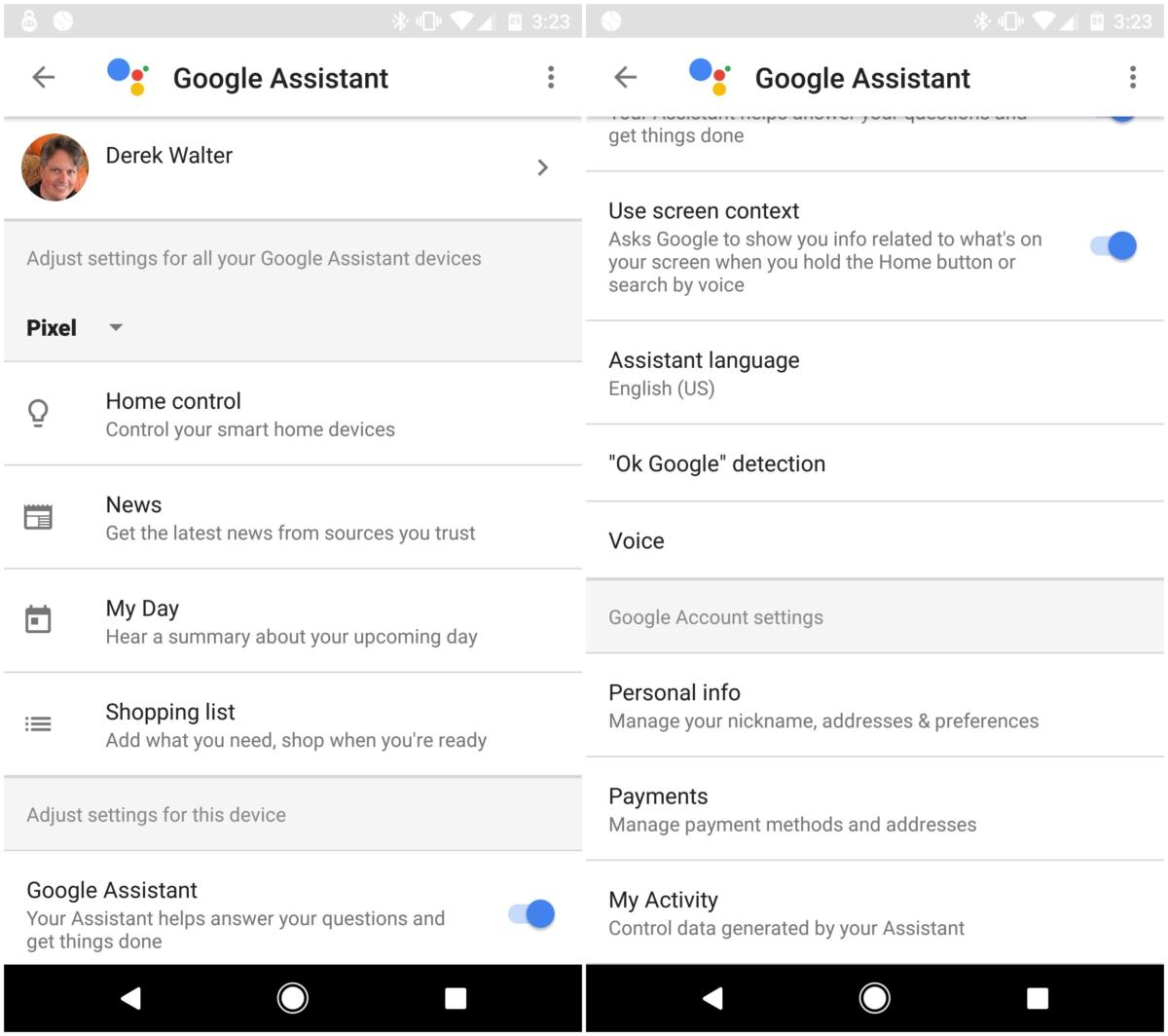The image depicts a website displayed side by side, showing identical elements in both instances. The top portion of each page features a light gray banner adorned with several icons, including a round padlock, a circular icon, a Bluetooth symbol, a cell phone indicating vibration, a Wi-Fi symbol, a cellular signal strength icon, and a battery status icon. The battery indicator displays a charge level of 3:23, consistent across both sides.

Beneath the banner on each side, there is a back arrow followed by colorful round circles in blue, green, red, and yellow, alongside the text "Google Assistant" in black with capitalized initials "G" and "A." Each side also features three vertical dots positioned on the right.

On the left page:
- There is a user's profile picture accompanied by the name "Derek Walter."
- Below this, a gray banner reads, "Adjust settings for all your Google Assistant devices."
- Further down, it lists various options such as "Pixel," a drop-down arrow, "Home Control," "News," "My Day," and "Shopping List."
- Another section indicates, "Adjust settings for this device."
- The "Google Assistant" option is shown with its toggle turned on.

On the right page:
- The display is partially cut off from the banner.
- It reads, "Get things done," followed by "Use screen context," with the toggle turned on.
- It lists "Assistant Language" set to "English (U.S.)."
- Options for "OK Google detection" and a section for "Google Voice or Google account settings," including "Personal Info," "Payments," and "My Activity."

Overall, the image captures a detailed view of two similar website interfaces focused on various settings and functionalities related to Google Assistant.